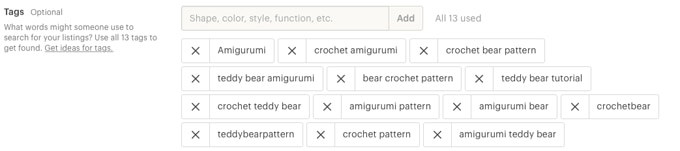The image features a user interface designed for optimizing search tags on a white background. Prominently highlighted is the phrase "tags optional," in bold text. Below this are instructions prompting the user on selecting keywords to enhance the visibility of their listings, ending with a question mark. The interface encourages utilizing all 13 tags to maximize discoverability. A search bar urges users to input various descriptors including shape, color, style, and function. Adjacent to the search bar, an underlined "get ideas for tags" link is also visible. 

Flanking the right side of the layout are a series of rectangular text boxes that include potential keywords: "crochet," "bear pattern," "bear crochet pattern," "teddy bear tutorial," "crochet teddy bear," "crochet bear," "teddy bear pattern," "crochet pattern," "amigurumi teddy bear," "amigurumi," and "amigurumi bear," "amigurumi pattern." To the left, there's a square marking the area to advance to the next step. An "add" button suggests the capability to input additional tags.